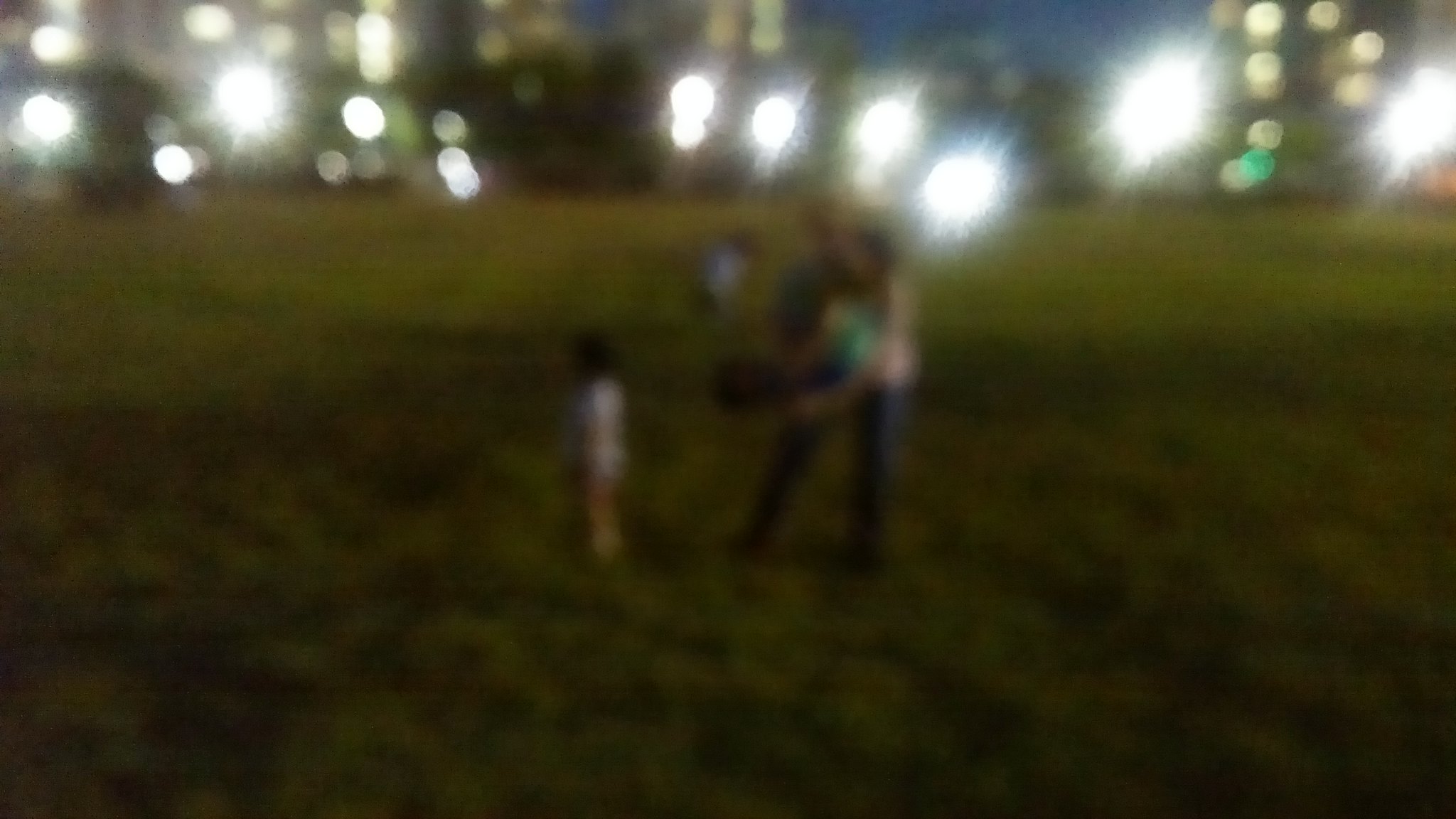An outdoor color photograph taken at night captures a dark, out-of-focus scene. In the foreground, there is a large grassy field that appears slightly inclined from the right to the left. Central to the image is a family group: a young child with black hair, dressed in a white shirt and brown pants, stands facing left. Behind this child are two adults; one crouched over, wearing a green shirt, and another standing behind, clad in a pink top and green pants. Adding to the complexity, there is possibly another adult dressed in blue jeans and a blue shirt, with indistinguishable features, and potentially holding another child. The upper third of the image shows a blurred cityscape with six or seven bright light glares spread across the background. The entire image is characterized by its excessive blurriness, making individual features and details indistinct.